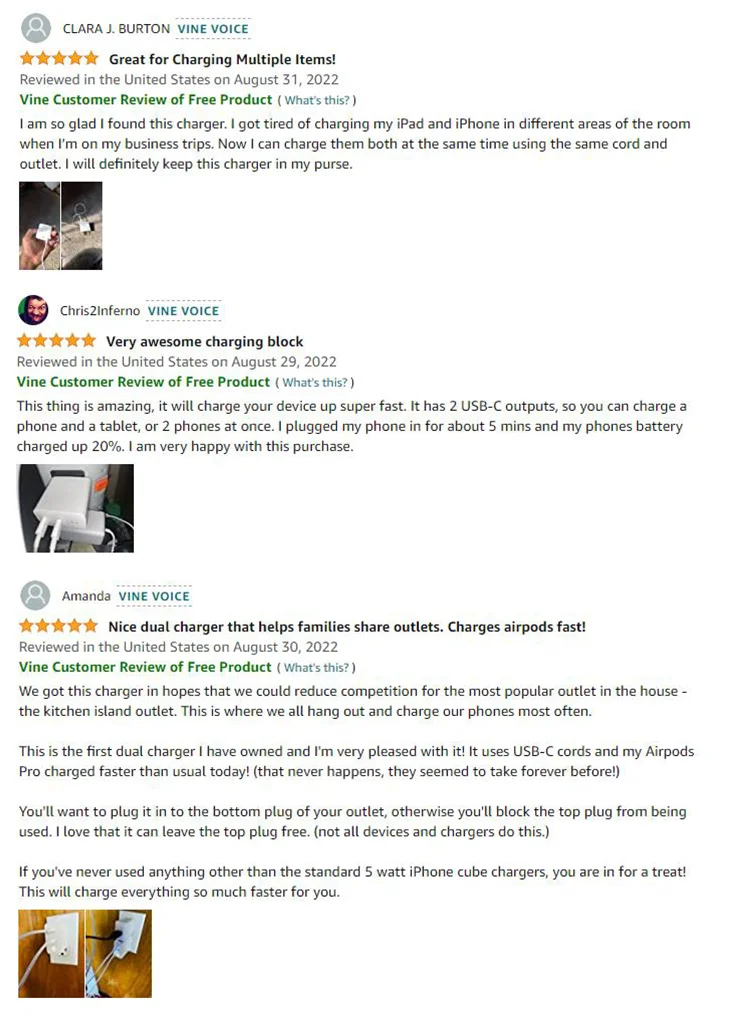### Amazon Product Reviews for Dual USB-C Charger

**Clara J. Burton**
- **Rating:** ⭐⭐⭐⭐⭐
- **Headline:** Great for Charging Multiple Items
- **Review:** "I am so glad I found this charger. I got tired of charging my iPad and iPhone in different areas of the room when I'm on my business trips. Now I can charge them both at the same time using the same cord and outlet. I will definitely keep this charger in my purse."
- **Photos:** 
   1. Photo of the dual USB-C charger plugged into a wall outlet.
   2. Close-up of the charger showing its dual ports.
- **Additional Information:**
  - **Reviewer:** Vine Voice
  - **Tagline:** Vine customer review of free product

**Chris2Inferno**
- **Rating:** ⭐⭐⭐⭐⭐
- **Headline:** Very Awesome Charging Block
- **Review:** "This thing is amazing. It will charge your device up super fast. It has two USB-C outlets so you can charge a phone and a tablet or two phones at once. I plugged my phone in for about five minutes and my phone battery charged up 20%. I am very happy with this purchase."
- **Photo:** 
  1. Image showing the charger in use with two devices connected.
- **Additional Information:**
  - **Reviewer:** Vine Voice
  - **Tagline:** Vine customer review of free product

**Amanda**
- **Rating:** ⭐⭐⭐⭐⭐
- **Headline:** Nice Dual Charger That Helps Families Share Outlets. Charges AirPods Fast.
- **Review:** "We got this charger in hopes that we could reduce competition for the most popular outlet in the house, the Kitchen Island outlet. This is where we all hang out and charge our phones most often. This is the first dual charger I have owned and I'm very pleased with it. It uses USB-C cords and my AirPods Pro charge faster than usual today. That never happens. They seem to take forever before. You'll want to plug it into the bottom plug of your outlet otherwise you'll block the top plug from being used. I love that it can leave the top plug free. Not all devices and chargers do this. If you never used anything other than the standard five-watt iPhone tube chargers, you are in for a treat. This will charge everything so much faster for you."
- **Photos:**
   1. Image of the charger being used on the Kitchen Island outlet.
   2. Close-up of the charger connected to an AirPods Pro case.
- **Additional Information:**
  - **Reviewer:** Vine Voice
  - **Tagline:** Vine customer review of free product